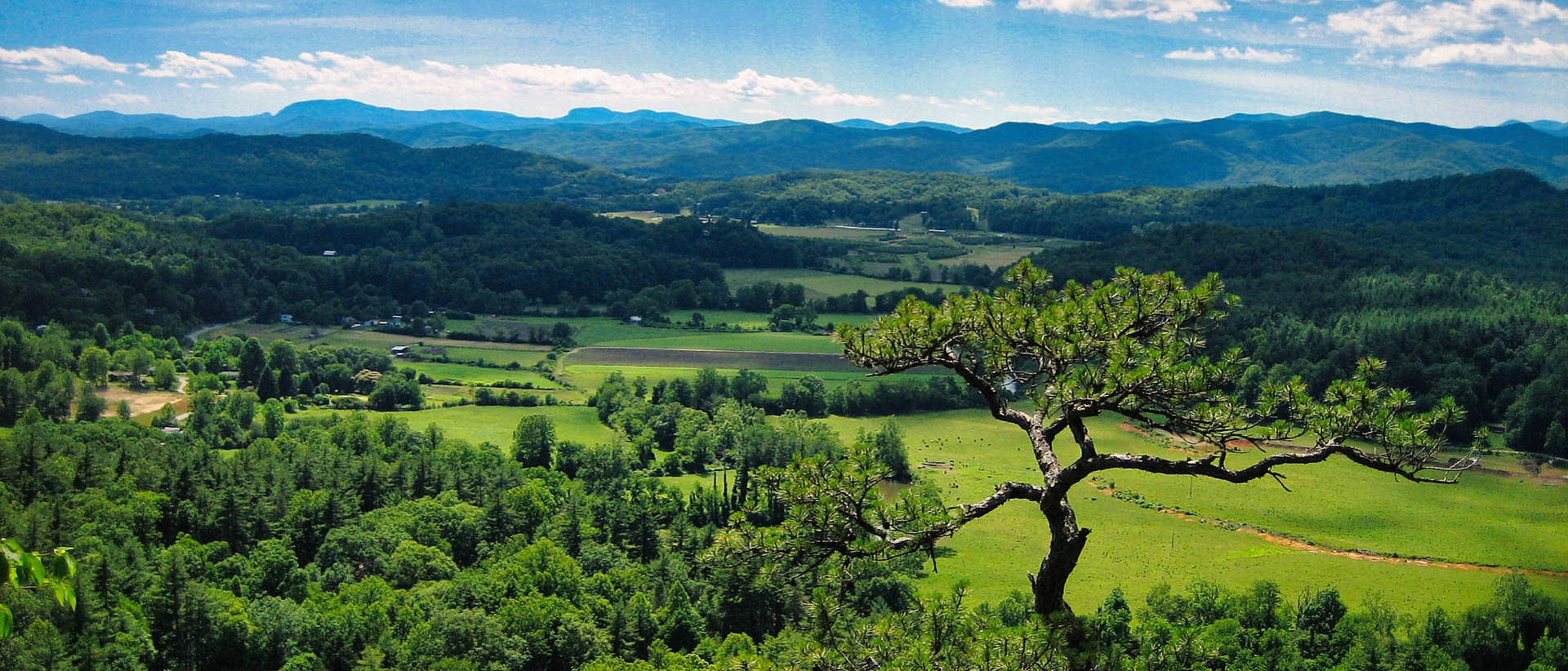The photograph captures a breathtaking panoramic view from atop a hill overlooking a lush, green valley. The scene is dominated by verdant fields of grass interspersed with numerous trees, creating a tapestry of varying shades of green. Central to the foreground stands an ancient, withered tree with three prominent branches adorned with small green leaves. 

Further into the distance, the valley transitions into a dense forest that stretches towards a formidable mountain range under a blue sky dotted with fluffy white clouds. The mountains, tinged with gray and green from the mix of rock and shrubbery, form a majestic backdrop to the expansive landscape. 

The shot also reveals a narrow country road cutting through parts of the valley, suggesting rural habitation, though no houses are distinctly visible. Some areas hint at farmland. The late afternoon sun casts long shadows across the valley from left to right, adding depth and contrast to the vibrant scene. The photograph eloquently captures the tranquility and immensity of the landscape, from the towering central tree to the distant mountain horizon.